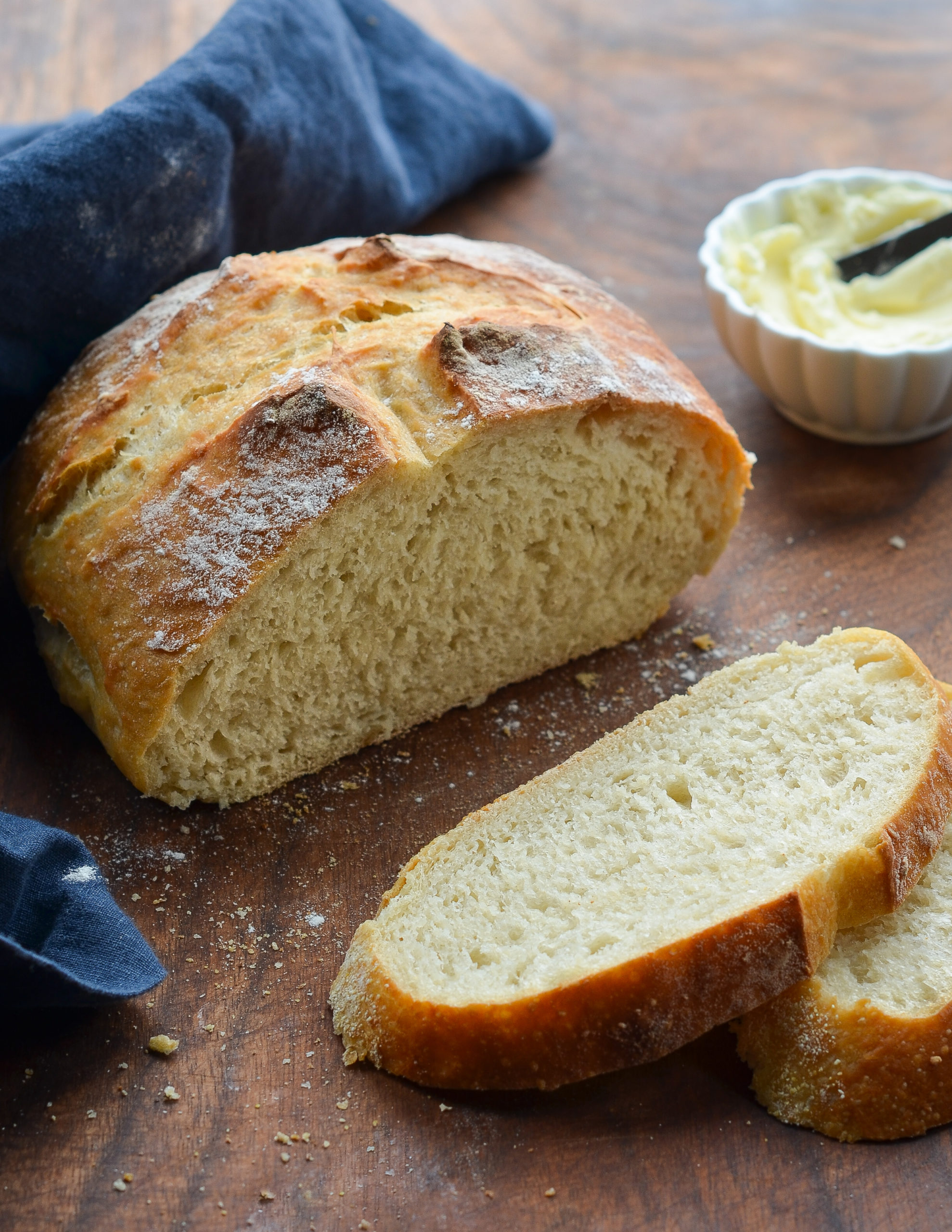In this detailed photograph, a freshly baked, small, round loaf of artisanal bread is prominently displayed on a wooden countertop. The loaf, which has a high, gently domed shape reminiscent of Italian bread, has been partially sliced. Two slices are placed one on top of the other in front of the loaf, revealing its airy yet dense texture. Surrounding the bread are scattered breadcrumbs and flour, accentuating its rustic quality. Behind the loaf lies a crumpled, midnight blue napkin, suggesting it was used to handle the hot bread straight from the oven. To the right of the loaf sits a small, fluted white china bowl containing softened butter and a knife, perfect for spreading onto the bread. The loaf's beautiful, dark brown crust adds to its delicious and inviting appearance, making it ideal for both everyday meals and fancy dinners.